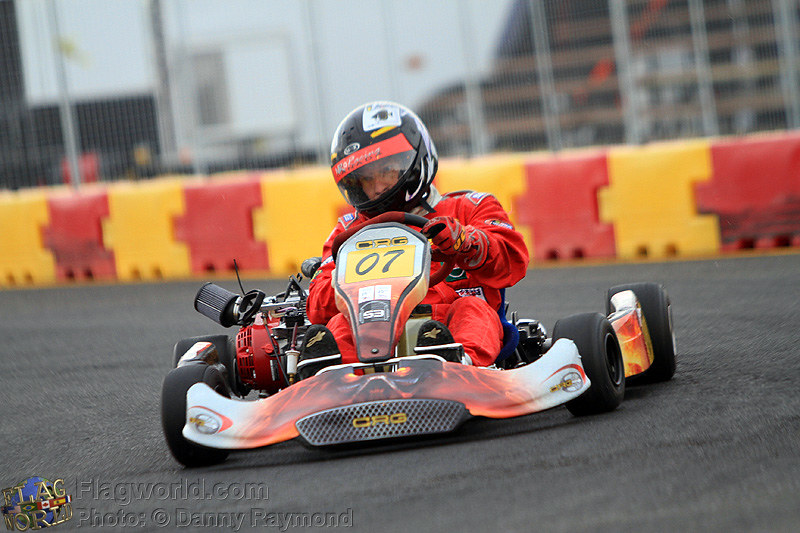The image captures a go-kart driver speeding towards the camera on a gray racetrack. The go-kart, bearing the number 07 prominently on the steering wheel and featuring white and red colors with airbrushed flames on the paneling, sits low to the ground and exudes a sense of speed and agility. The driver, clad in a flame-retardant red race suit, red gloves, and a black helmet adorned with red and white decals and a clear visor, focuses intently ahead. Surrounding the track is a safety wall painted in yellow and red, topped with fencing that partially obscures the wooden stadium seats in the background. At the bottom of the image, a watermark reads "hagworld.com, photos copyright Danny Raymond."